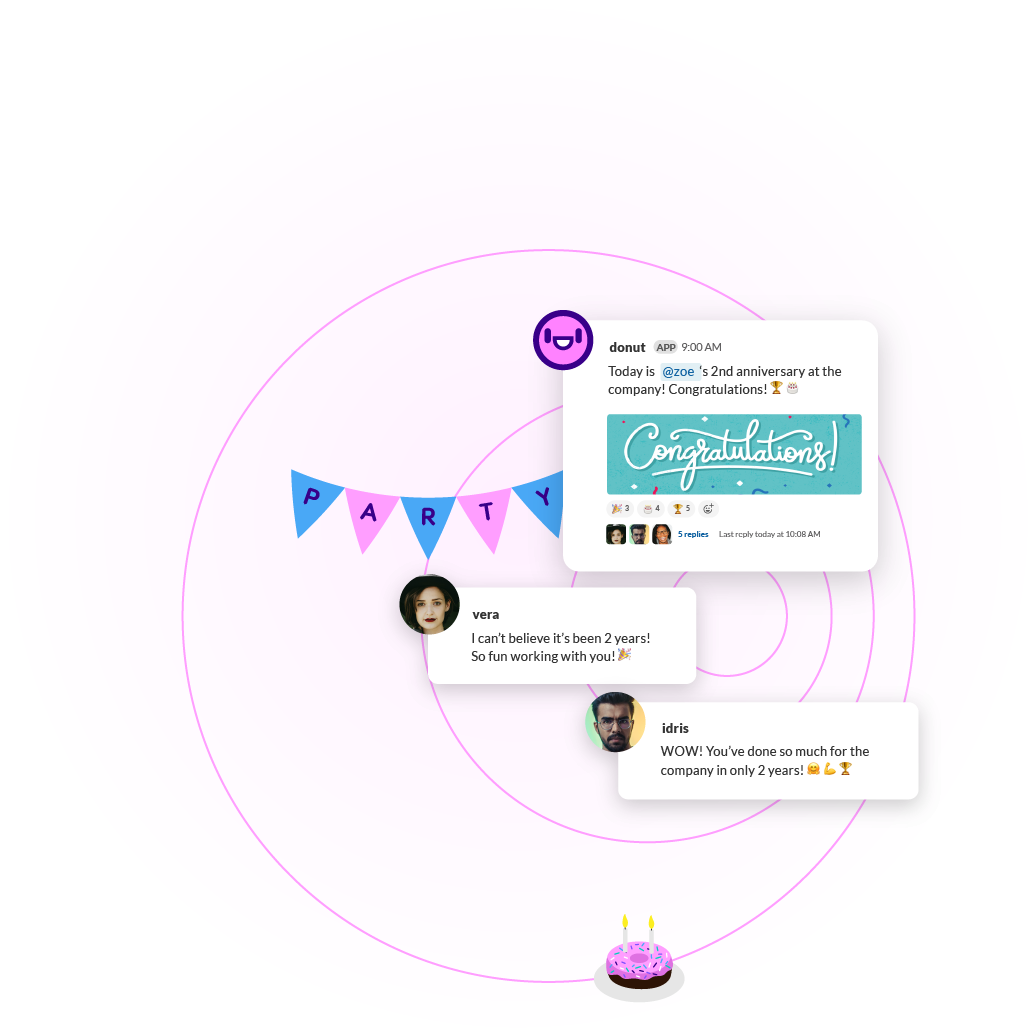The graphic showcases a celebratory theme within an internal company messaging system, featuring vibrant visual elements. Dominating the background is a large, purple circle outline, with several smaller concentric circles situated slightly to its right. In the center of this arrangement is a whimsical flag banner, adorned in hues of blue and pink, spelling out the word "PARTY" with each letter on an individual pennant.

In the top-right corner, an image celebrates an employee's second anniversary at the company. This section includes a congratulatory message and a banner reading "Congratulations." Below this, three profile pictures of colleagues who have interacted with the celebratory comet are displayed.

Offset to the left within the center of the graphic, a comment by a woman named Vera reads, "I can't believe it's been two years. So fun working with you." To the right, another comment highlights the employee's contributions, stating, "Wow, you've done so much for the company in only two years." Along the bottom-right edge of the primary circle, a delightful donut cake graphic adds a festive touch to the composition.